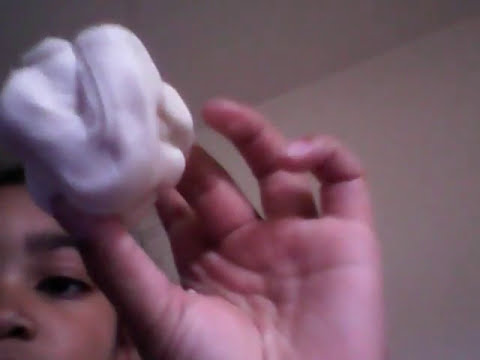In this image, a young woman with dark hair and brown skin is holding up a soft, white, crumpled object in her left hand, positioned between her thumb, middle finger, and ring finger. Her hand, with visible palm lines, is raised in the bottom left corner of the frame, revealing a slightly bent pinky. The scene is somewhat blurry, capturing only part of her face above her lip, revealing one dark eyebrow, one eye, a nostril, and her dark hair. The background shows an indoor setting, likely a room with eggshell or off-white walls and ceiling, adding to the intimate, spontaneous feel of the image, which may have been taken in a selfie style or with a webcam.